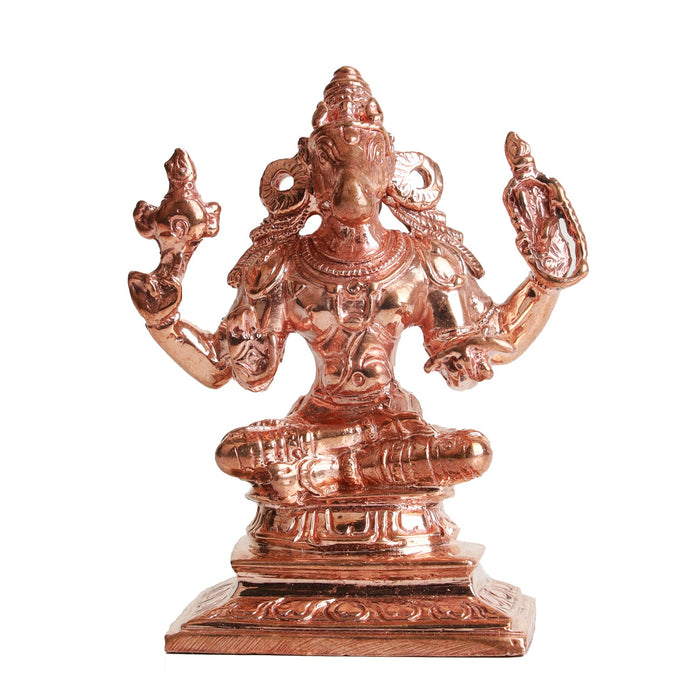The image portrays a pinkish-brass colored statue, representing a deity seated cross-legged on a pedestal. The figure resembles a yogi adorned in elaborate jewelry, including large circular earrings with tassels, ornate necklaces, bracelets, and a lower body covering, yet appears shirtless. The face is anthropomorphic, blending features of a goat, indicated by twirling horns, and possibly a bird-like visage. The deity is depicted with raised arms, each hand holding an unidentified object, possibly a rope or religious symbol. The statue has an oriental, possibly Hindu or Eastern, aesthetic, accentuated by its vibrant gold armor-like adornments with a distinctive pinkish-red hue, all set against a plain white background.